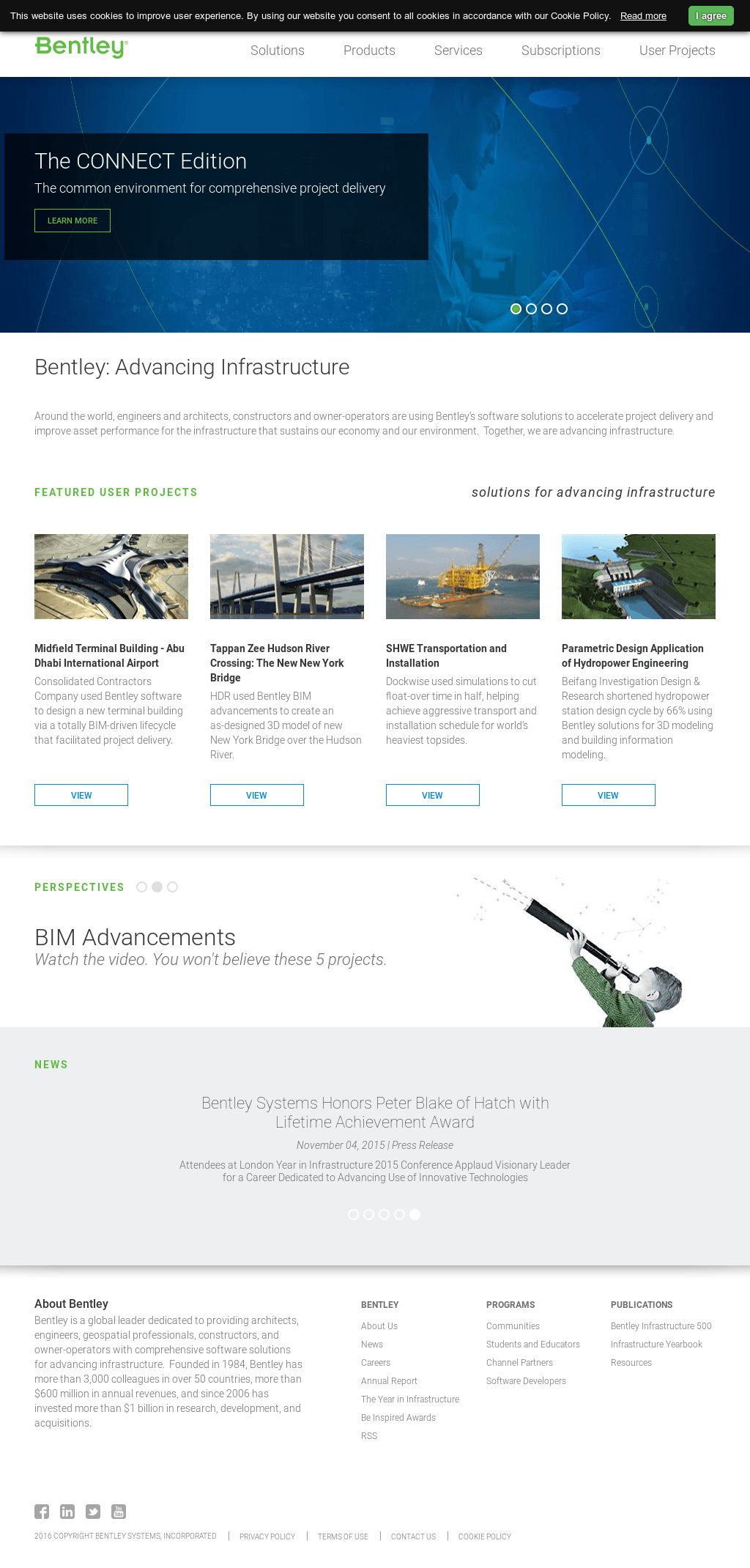The image depicts a detailed screenshot of a web page, which appears to be divided into multiple sections. 

At the very top, there is a black bar containing illegible text, likely due to its small font size. Directly below this bar, the iconic green Bentley logo is prominently displayed. Underneath the logo is a navigation menu with the following items listed: Solutions, Products, Services, Subscriptions, and User Projects.

The next section features a wide blue rectangle stretching across the entire width of the screen. Inside this blue rectangle is a smaller black rectangle that contains the text "The Connect Edition." Although the full text is unreadable, it mentions "project delivery." Below this black rectangle is a green button labeled "Learn More."

The rest of the page has a white background. The text "Bentley Advancing Infrastructure" is visible at the top of this section, followed by a paragraph that is too small to decipher. Beneath this paragraph is a heading in green that reads "Featured User Projects." To the right, written in black, is another heading, "Solutions for Advancing Infrastructure."

At the bottom of the page, there are four photos displayed in a row. The first image captions something related to a terminal building, though it's not fully readable. The second image depicts what appears to be a bridge. The third image shows a large crane, and the fourth and final image features a building with a swimming pool. Below each photo, there are buttons whose purposes are not specified in the description.